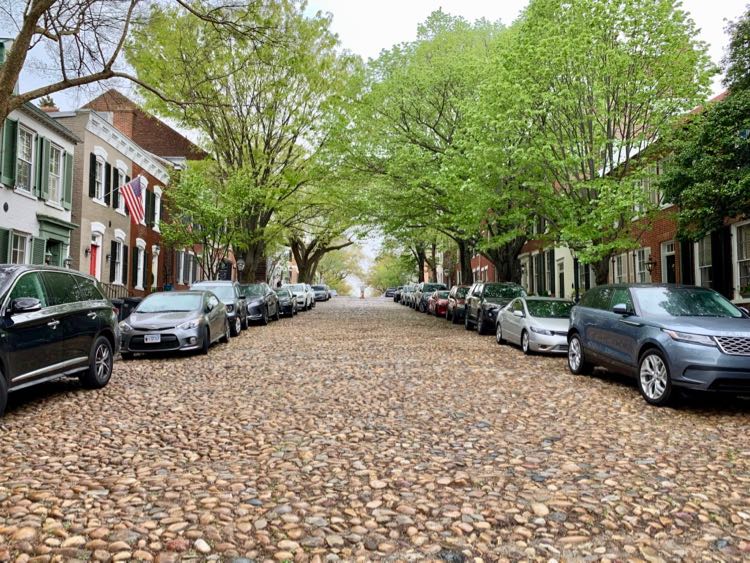This image captures a tree-lined, densely packed neighborhood street composed entirely of cobblestones extending far into the distance, creating a picturesque vanishing point. Both sides of the one-way street are flanked by parallel-parked cars, all uniformly facing towards the camera. The houses lining the street are predominantly two-story units, with no visible front yards, suggesting a close-knit urban community. Most of the homes on the right side exhibit a uniform brownish hue, while a notable red two-story house on the left, adorned with a brown awning and an American flag, stands out. Tall trees, numbering at least four, punctuate the middle of the block, their canopies contributing to the lush, green overhead. The absence of moving vehicles enhances the serene, almost timeless quality of this cobblestone street scene.